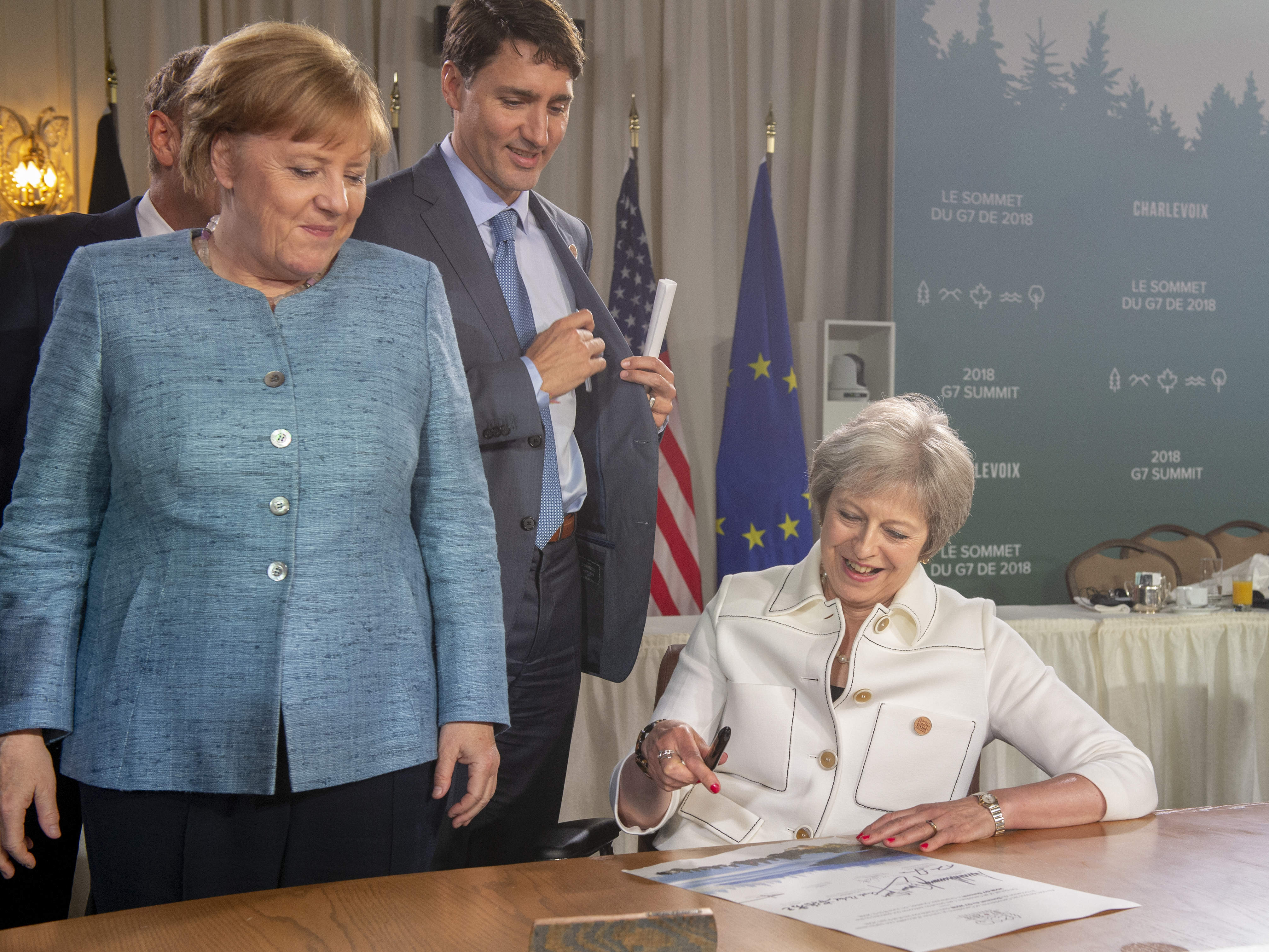In this photograph, taken at the 2018 G7 Summit, a group of international leaders is gathered in what appears to be a conference hall. Central to the scene is an older woman with short gray hair, sitting at a light brown wooden table. She is wearing a white cardigan with brown buttons and is smiling as she signs a large poster with a pen in her right hand. To her right stands a woman with short light brown hair, identified as the former German Chancellor Angela Merkel. Merkel is wearing a blue buttoned-down cardigan with silver buttons and is looking down at the signing woman with a slight smile. Beside Merkel, a man believed to be the Canadian Prime Minister, Justin Trudeau, is visible. He is a white male with short dark hair, dressed in a gray suit with a blue tie. Trudeau is holding a rolled-up piece of paper in his left hand and appears to be placing a pen or another small item into his jacket pocket with his right hand, all while also focusing his attention on the woman at the table. Behind these individuals, several national flags can be seen, including the American flag and a blue flag with yellow stars, likely the European Union flag. The background features long gray curtains and a poster with trees and white text, further contextualizing the setting as an international summit. Additionally, a light can be seen in the top left corner, and another table with a white tablecloth and some objects like a glass of orange juice are present, indicating a few more details of the room's furnishings and the event's formal environment.